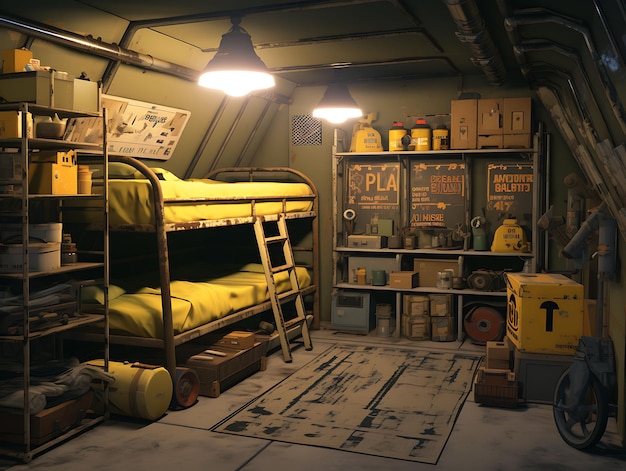The image vividly captures the interior of a compact underground bunker, draped in a muted palette dominated by greenish-gray tones enveloping the entirety of its walls and floor. On the left side, a set of meticulously placed bunk beds features bright yellow bedding, adding a stark contrast to the otherwise somber ambiance. Attached to the bunk beds, a small ladder offers access to the upper bunk. Surrounding the bunk beds, shelves—constructed from industrial metal—are laden with an assortment of survivalist gear, including rows of metal containers and boxes of various colors like yellow, black, and gray. Some of these boxes bear inscriptions in an unfamiliar alphabet, possibly Russian. The ceiling hosts two slightly off-centered, bare bulb lights, casting a dim yet essential glow over the scene. The floor is partially covered by a dark brown rug, which rests atop the brownish tiles, adding a touch of warmth to the stark environment. Notably, the bunker lacks windows, reinforcing the isolated nature of this subterranean space.